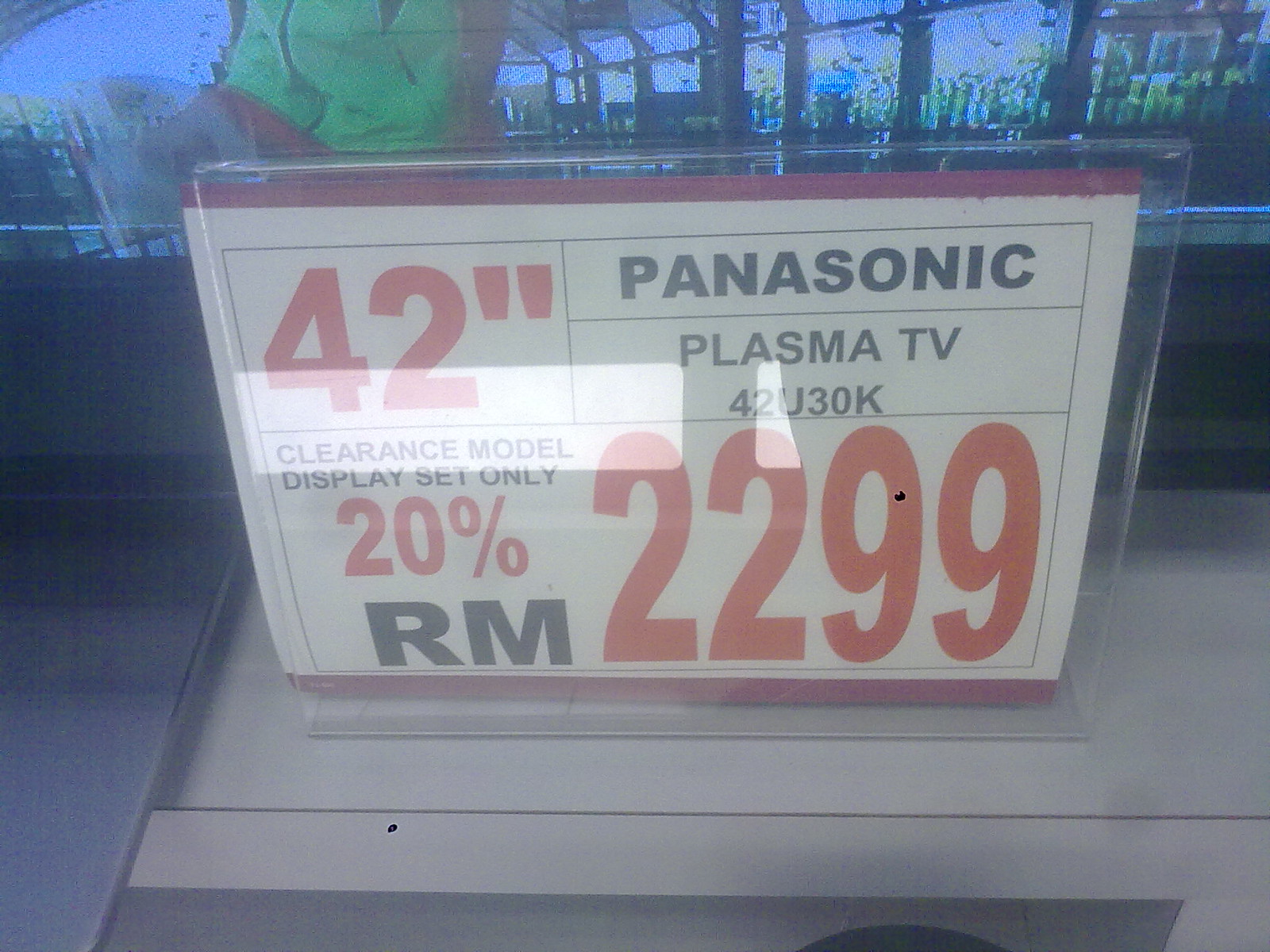This detailed image appears to be a full-color photograph taken through a storefront window, likely of an electronics store. The focal point is a small sign encapsulated in a plastic stand, which is centered in the square frame of the photograph. The sign advertises a 42-inch Panasonic Plasma TV, model 42U30K, offering a clearance discount of 20%, bringing the price down to RM2,299 (Malaysian Ringgit). The sign's text is prominently displayed in red, black, and white fonts. The surrounding colors include hints of blue, green, and grey. Behind the sign, it's difficult to discern precise details, but it appears to be the bottom part of a TV screen and a series of other electronics, most likely televisions, which are blurred due to the digital quality of the image and reflections from the storefront glass. Elements of outdoor structures are faintly visible at the top of the image, adding context to the setting. This photograph captures the essence of an older advertisement, highlighting a technology that has since become outdated with the discontinuation of plasma TVs.